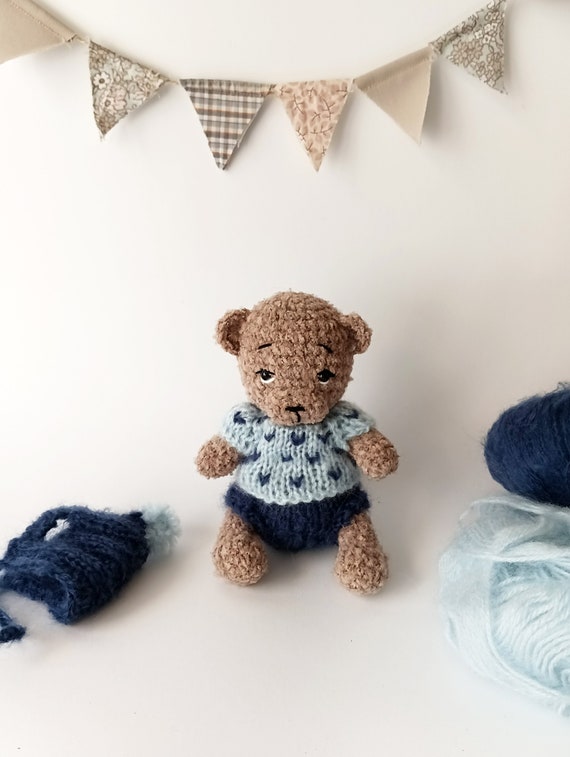This professionally taken photograph, likely intended for a magazine, centers on an intricately hand-knit teddy bear set against an off-white background. The bear itself is brown with black eyes, donning a light blue sweater accented with darker blue patches and matching dark blue knitted shorts. The bear sits serenely on an off-white surface. Positioned to the left of the bear is a small knitted item, possibly a hat or scarf made from dark blue yarn. To the right, skeins of both dark blue and light blue yarn, akin to the shades used in the bear’s attire, lay unwound. Dangling above the bear is a string of six triangular patches, resembling party streamers, featuring a variety of patterns including floral designs and gradients of tan, brown, and off-white. The backdrop and surface share a harmonious creamish-white hue, enhancing the quaint and cohesive aesthetic of the scene.